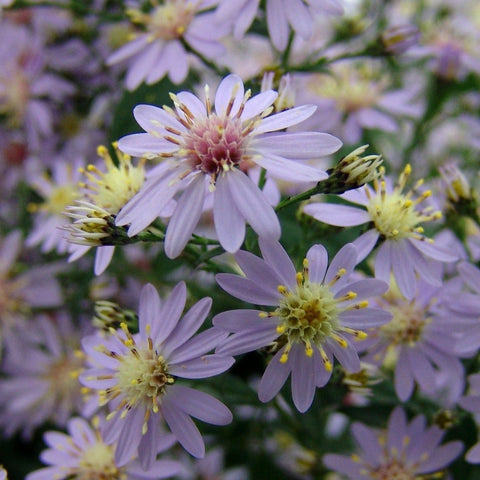This photograph features a close-up view of numerous pale lavender, daisy-like flowers set against a green background, likely foliage or stems. The flowers, similar in appearance to daisies, display soft lilac petals with centers that vary between yellow and purple. The highest flower in the very center of the photo distinctively has a purple center. The image is taken from a top-down perspective, allowing a clear view of the intricate details within the blooms. The focal point centers on about five prominently sharp flowers in the foreground, while a multitude of additional flowers stretches out into a more blurred background. Overall, the visual captures the beauty and abundance of the blossoms, creating a charming and detailed depiction of the floral scene.